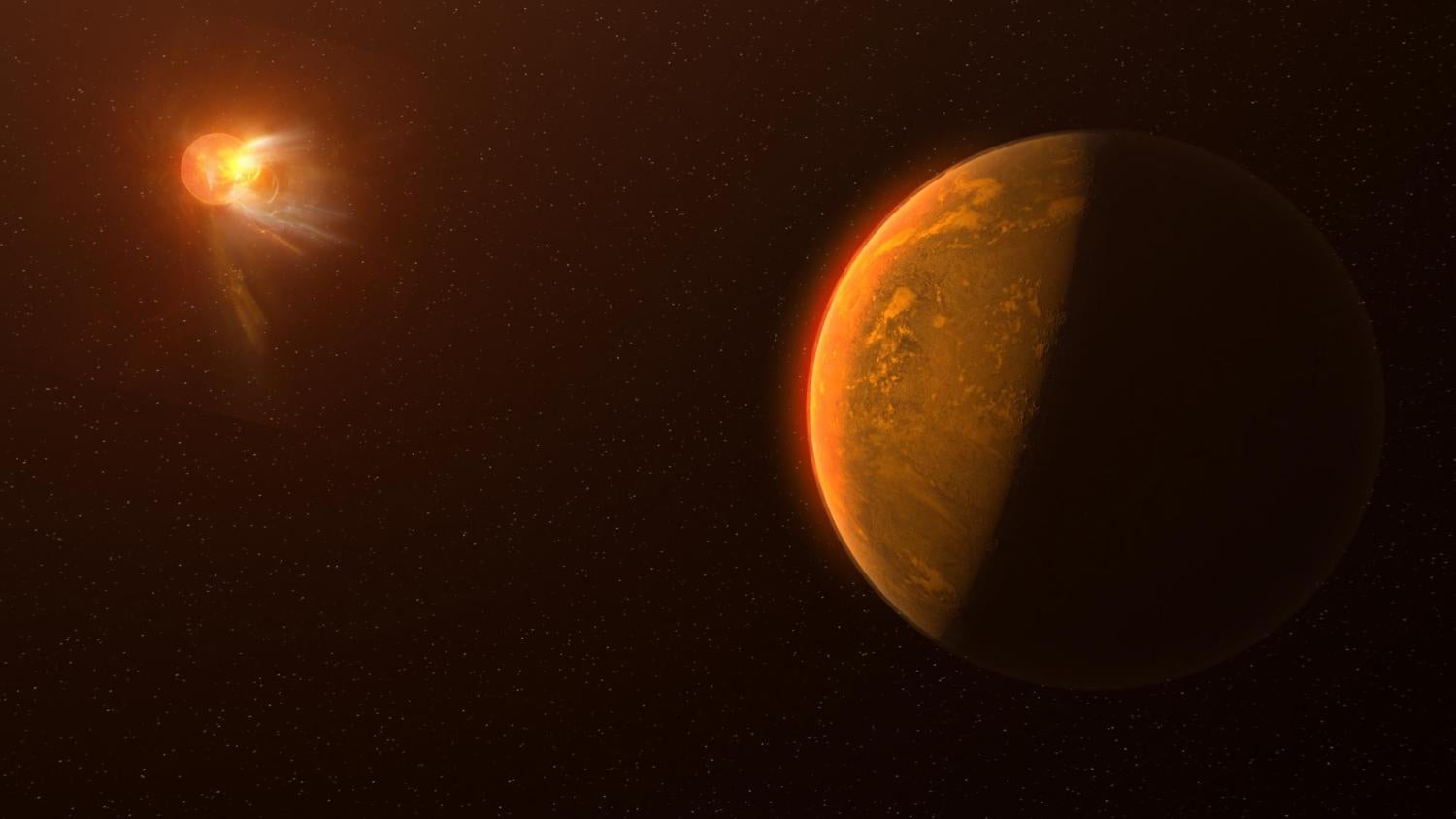This digital illustration portrays an otherworldly scene in outer space. On the right side of the image, there's a partially illuminated planet, possibly Earth, though it appears more reddish-orange, hinting at an alien or altered version of our planet. The left half of this planet is engulfed in a deep shadow, while the illuminated portion glows in hues of red and orange, suggesting it's being affected by intense solar activity.

On the far left side of the image, an orb resembling our Sun emits powerful yellow and orange solar flares or cosmic rays, streaking across the dark space towards the planet. These energetic beams seem to be the source of the vivid illumination on the planet's surface. The background of the image remains a stark black, peppered with white dots representing distant stars, contributing to the sense of a vast and mysterious cosmos. This digitally created photo, with its dominant black, orange, and yellow palette, appears to be designed for astronomy visualization or perhaps as an artistic render for a game, capturing a dramatic celestial event.